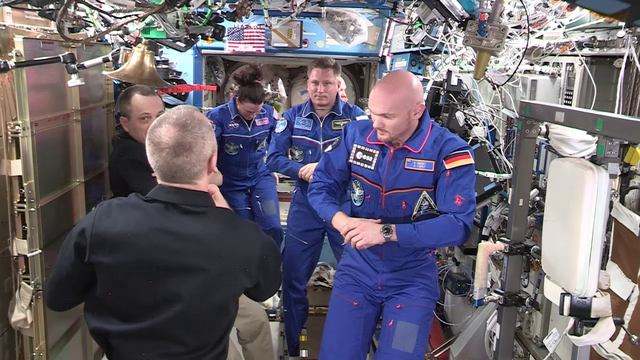The image is a horizontal landscape color photograph capturing the interior of what appears to be the International Space Station or a similar space shuttle environment. The tight, compact space is cluttered with scientific equipment, wires, straps, and various metallic and plastic components hanging from the walls and ceiling. Prominently displayed on one of the blue walls in the background is a small American flag. The photograph features five astronauts, identifiable by their blue attire adorned with various patches and insignias. 

Three astronauts stand on the right side. The one closest to the camera is bald with a small beard and sports a German flag on his left shoulder. Next to him is a woman with dark hair tied back, and beside her is a man with brownish hair, both in blue jumpsuits that feature white or red trims, zippers, and several patches, although the specific details on the patches are not clearly visible. These blue jumpsuits are full-body, with collars and long sleeves.

On the left side of the frame are two men in black shirts and beige or gray pants. One of these men has his back to the camera, while the other faces towards the right side of the image. Both men appear to have short hair and are ethnically white. All five individuals seem to be experiencing zero gravity, as evidenced by their slightly bent legs and the way they hold their hands clasped in front of them to stabilize their positions.